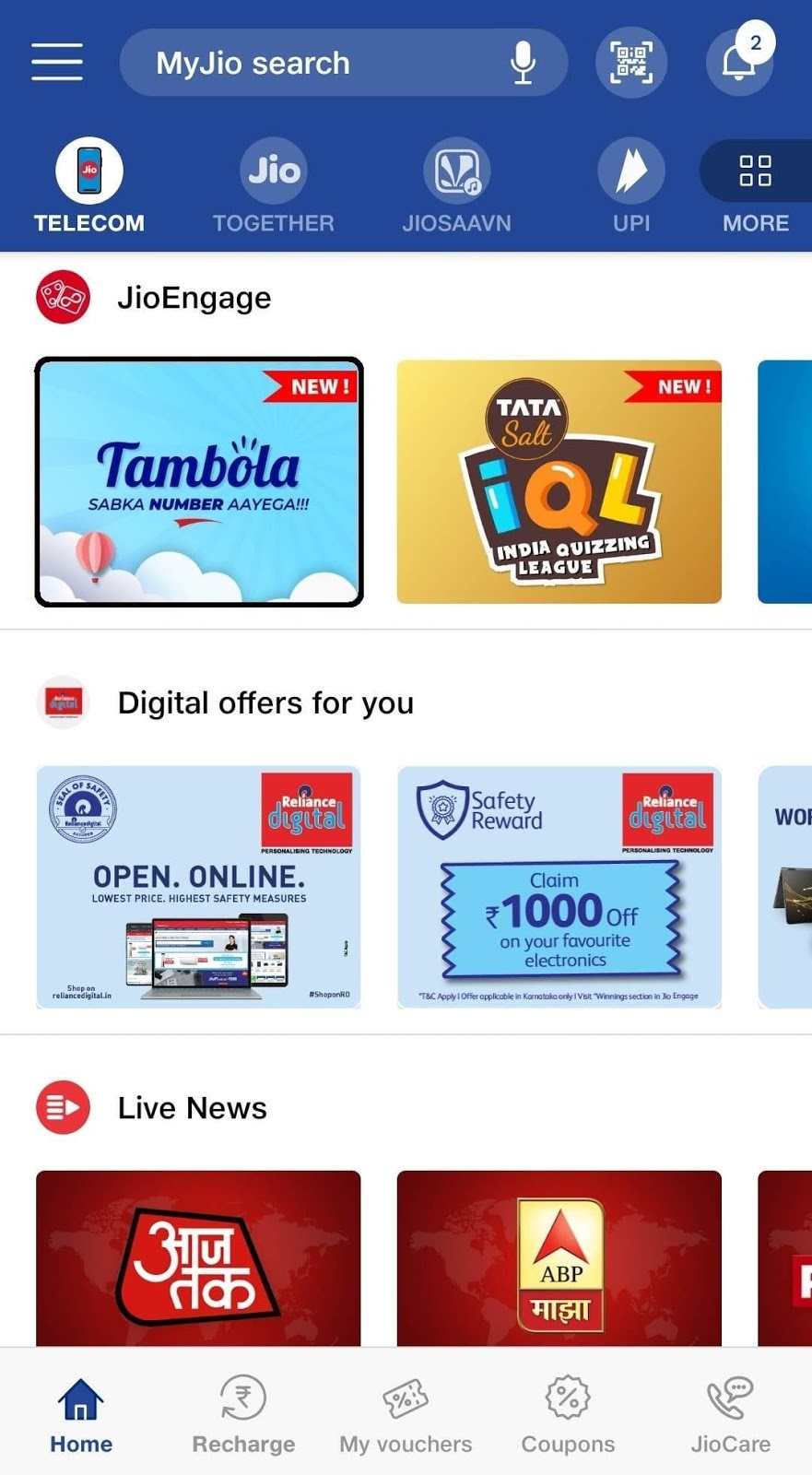This is a detailed caption for the given image description:

---

This is a smartphone screenshot of the MyGeo or GeoEngage website. The website's icon is depicted as two dice, one displaying the number four and the other displaying the number two, both enclosed within a red circle. At the top of the screen, there is a blue border featuring a hamburger menu on the left. To the right of the menu is a search box titled "MyGeoSearch," which includes a microphone icon at the end. Next to the search box are icons for QR code scanning and notifications, with the notification icon indicating two unread messages.

Immediately below the blue border, there are several icons arranged horizontally. The first icon represents telecom services and is depicted with a smartphone graphic. The second icon is labeled "Geo," followed by an icon for "Together." Next is an icon suggesting a music service named "GeoSaavn," indicated with the text "G-I-O-S-A-A-V-I-N." To its right, there are two white arrows in a blue circle labeled "UPI." A "more" icon, represented by four squares, is also present.

Below this horizontal row of icons is the main GeoEngage icon, again depicting dice. Underneath, there are sections labeled "New," showcasing products such as "Tambola," "Sabka Number I-E-K-A," and "Tata Salt IQL - India Quizzing League," both marked with "new" banners. Further down, a section titled "Digital Offers for You" is displayed, featuring online sales of computers or laptops. To the right is a "Safety Reward," offering a chance to claim $1,000 off favorite electronics.

At the bottom of the screenshot, there is a row of icons related to navigation and additional services. These include a "Live News" icon, and two boxes containing text in an unspecified language. The first box has a red upward-facing arrow with the text "ABP" below it, followed by additional unreadable text in the same unknown language. Finally, the bottom row of icons includes: a "Home" icon (indicating the current section), a "Recharge" icon, a "My Vouchers" icon, a "Coupons" icon, and a "GeoCare" icon.

---